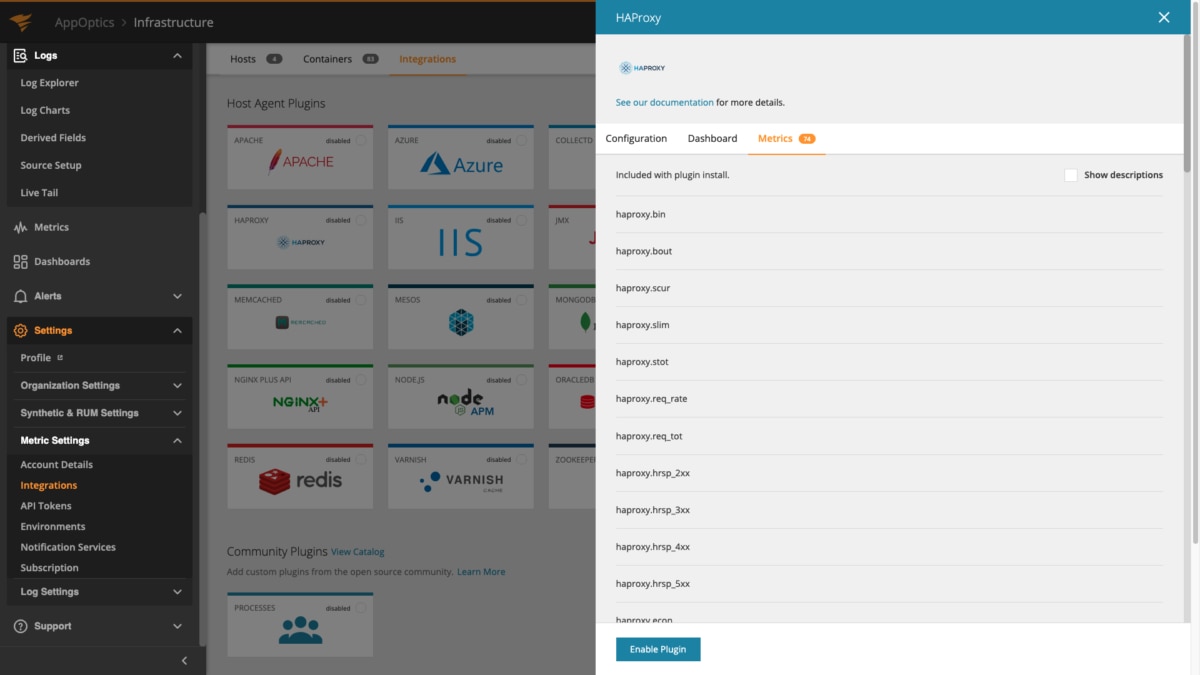Screenshot of Backend User Interface for Host Agent Plugins

In the foreground, a detailed screenshot captures the backend user interface of a software application. On the left side, a grey sidebar lists various navigation options. Adjacent to this, the main content area prominently displays a section titled "Host Agent Plugins." This section is organized into multiple rectangular tiles, each featuring distinct logos, with "Apache" and "Azure" appearing in the top row.

Additionally, a pop-up window is visible on the right side of the image. The window has a blue header bar with white text that reads "HAProxy." Below the header, the window is light grey and divided into three tabs: Configuration, Dashboard, and Metrics. The "Metrics" tab is currently selected, highlighted in orange, and underlined, indicating it is the active view.

This interface is instrumental for users seeking to monitor and optimize their system's effectiveness through detailed plugin management and metrics analysis.